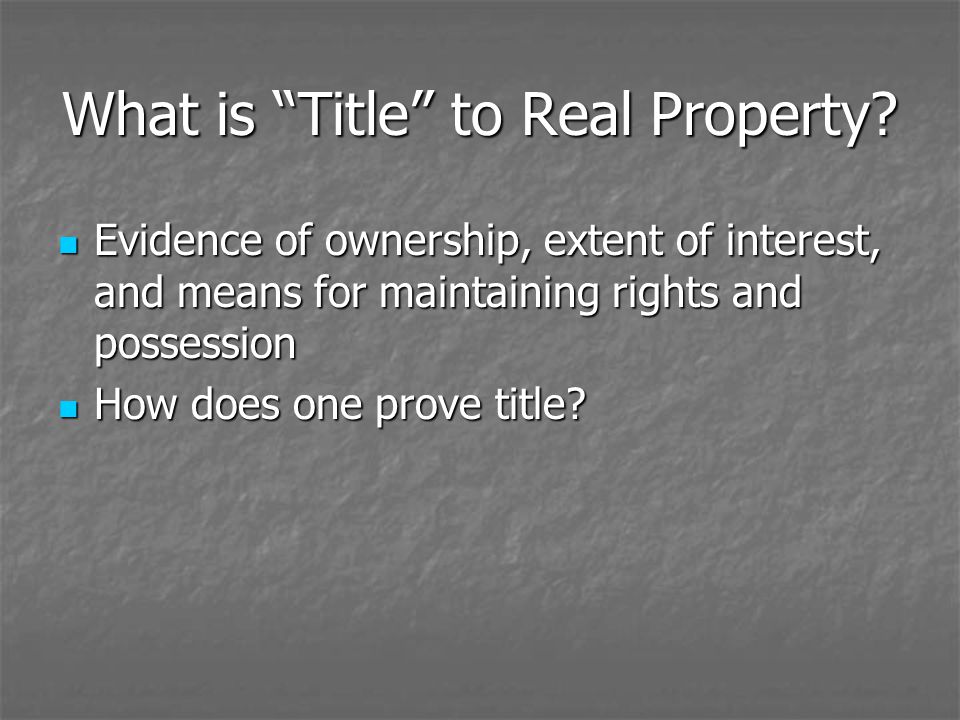The image depicts a presentation slide with a gray textured background, resembling crumpled paper that has been flattened out, with a darker shade at the top and bottom. The text is in white font, with a header that reads "What is 'title' to real property?" Below the title, there are two light blue rectangular bullets. The first bullet point lists "Evidence of ownership, extent of interest, and means for maintaining rights and possession." The second bullet point asks, "How does one prove title?" The slide appears to have originated from a computer program, such as PowerPoint.